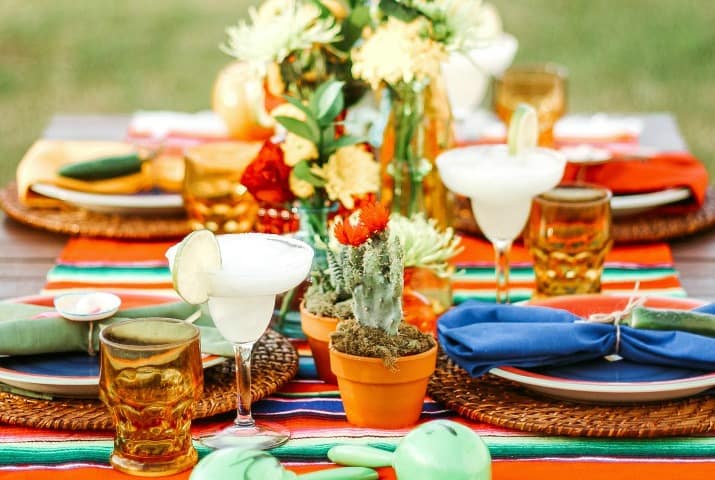This highly stylized and colorful image captures a close-up of a meticulously arranged picnic table setting, potentially inspired by a Cinco de Mayo or Southwestern theme. Dominating the scene is a vibrant table runner, primarily orange with accents of green and blue stripes, evoking a traditional Mexican blanket. The table itself, likely brown, hosts four intricately woven circular place settings, each topped with bold blue and red plates.

Situated at the center of the table are small potted blooming succulents, accompanied by an array of orange, yellow, and white flowers, adding a lively and natural touch. Each place setting is adorned with napkins in varying colors – yellow, red, blue, and sage green – which match the festive color scheme of the table runner. 

In front of each plate, there is a glass containing a fresh margarita, garnished with limes, enhancing the celebratory atmosphere. Additional glasses, possibly filled with water or other beverages, are also present on the table. The background of the image is blurred, drawing focus to the elaborate and thoughtfully designed table setting, making it resemble a scene from a high-end magazine or a themed event.